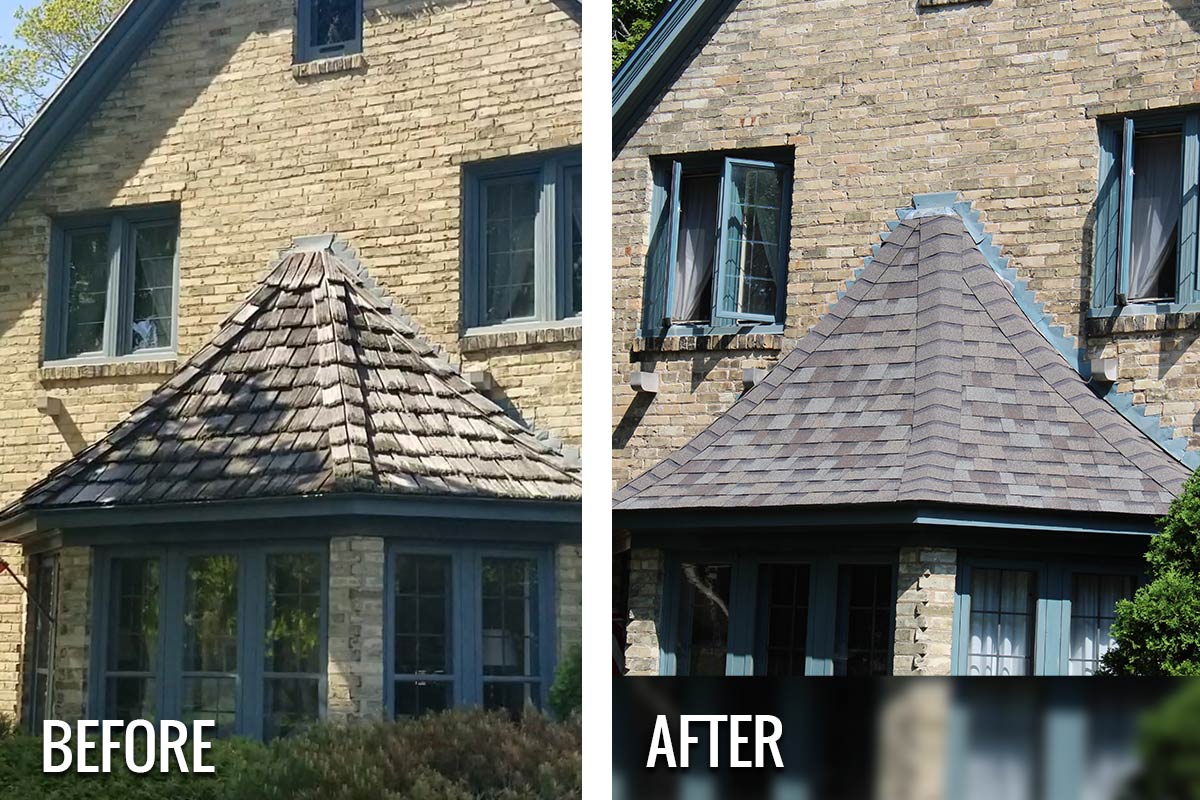This image showcases a striking before-and-after transformation of a red brick home, presented in a side-by-side, split-screen format. On the left, the "before" image reveals a weathered house with heavily worn wooden shingles on a protruding section with a small triangular roof. The shingles appear rough, discolored, and aged, and the yard is dotted with overgrown bushes. The windows, outlined in blue, look neglected. The "after" image on the right highlights significant improvements, including the replacement of old shingles with fresh, new, tar shingles, now neat and gray. The bricks appear cleaner, the windows have been painted a brighter shade of blue, and the surroundings look manicured, with overgrown bushes cleared away. Delicate light purple curtains adorn the now open windows, enhancing the fresh, revitalized look of the house.